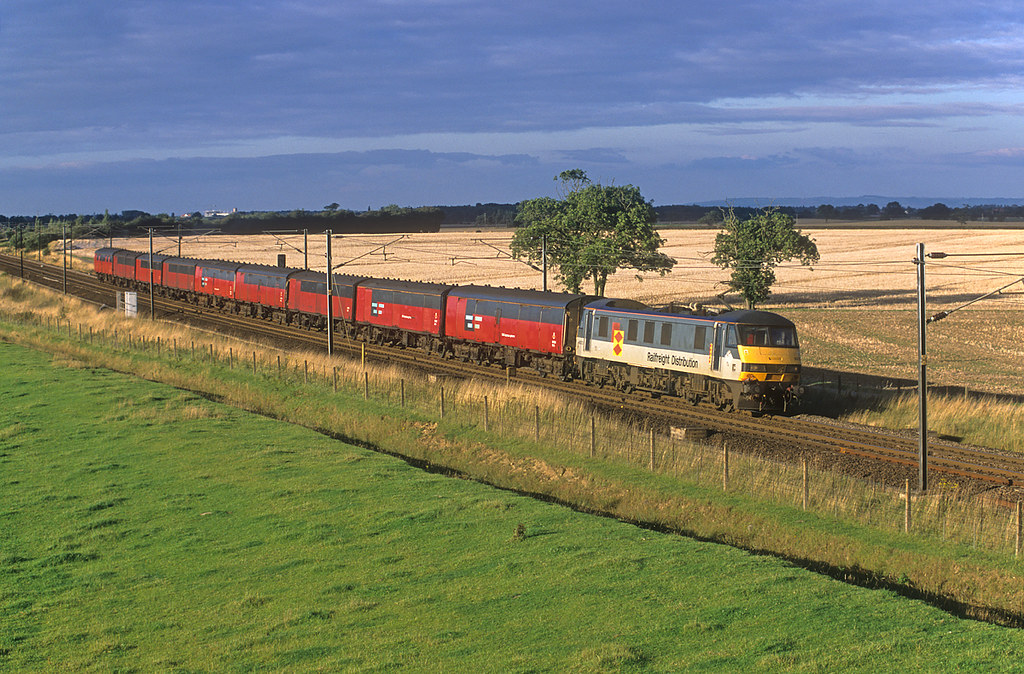The image depicts a vibrant countryside scene with a train traveling horizontally across the center. The foreground is dominated by lush, bright green grass, contrasted sharply against a fence running parallel to the railroad tracks. The red train, with its caboose adorned in white, yellow, and black, stands out vividly against the landscape. In the background, the grass shifts to a yellowish, tan hue, creating a striking contrast with the foreground. Notably, the middle field is dotted with a few trees, while a distant tree range marks the horizon, beyond which some mountains or hills can be seen. The sky is cloudy, painted in shades of dark and light blue, hinting at an evening or twilight hour with intriguing lighting and long shadows. Additionally, the train bears the text "rail freight distribution." The scene includes some fencing alongside the track and a few poles with possible electrical wires, indicating a practical countryside setting.